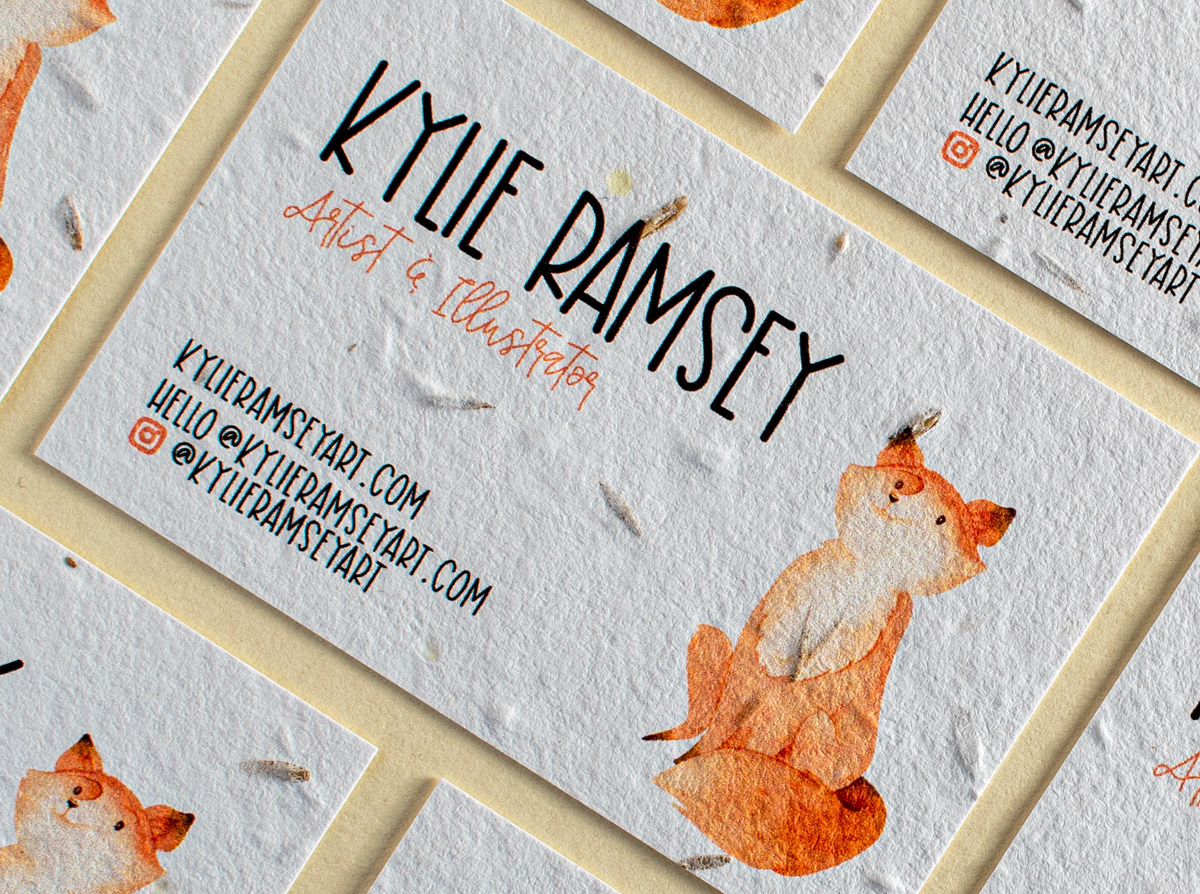This is a detailed top-down close-up image of a business card belonging to Kylie Ramsey, an artist and illustrator. The card is printed on a natural, rough-textured paper that appears to be embedded with flower seeds and boasts grainy divots reminiscent of old-school recycled material. The card is primarily dominated by large, bold capital letters stating "KYLIE RAMSEY." Beneath this, in elegant red cursive, it reads "artist and illustrator." Further information is provided below in black capital letters, including her website "KylieRamseyArt.com," her email "hello at KylieRamseyArt.com," and her Instagram handle "@KylieRamseyArt," presented alongside the Instagram logo. The right side of the card features a beautifully painted fox with orange and white fur, small black eyes, black-tipped ears, black-tipped legs, and a long, fluffy tail ending in a white tip. The card itself is displayed at an angle, approximately 30 to 40 degrees, extending from the upper left to the lower right, and seems to be framed by a plastic barrier. This framing effect is further emphasized by the staggered formation of repeated card designs in the background, akin to brickwork. Additional details include a gray background with beige rectangular outlines, and shapes of birds and leaves embossed into the paper.